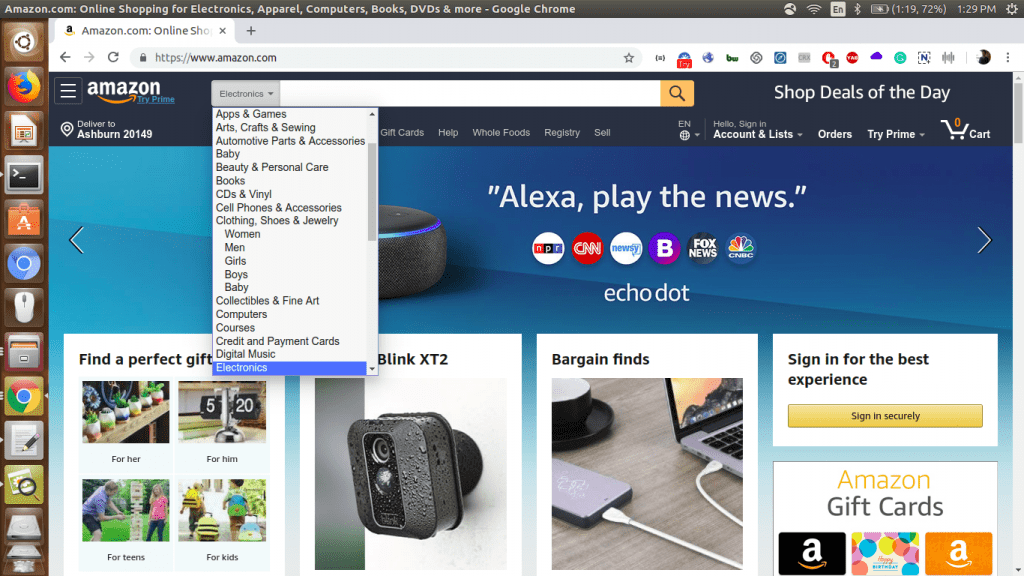This screenshot captures a typical Amazon.com homepage viewed on Google Chrome. At the top of the browser, the navigation bar indicates the website (Amazon.com) and is adorned with standard system icons such as Wi-Fi, Bluetooth, battery status, and the clock displaying 1:29 p.m. Underneath the address bar, only one tab is visible with the Amazon logo.

The Amazon webpage features a prominent search bar with a drop-down menu where the category "Electronics" is highlighted. Just below the drop-down menu, there is a banner image displaying an Amazon Echo Dot with the caption "Alexa, play the news." Navigation arrow buttons allow users to shuffle through additional promotional images.

On the left side of the page, there is a section dedicated to gift ideas labeled "Find the perfect gift for," accompanied by categories: her, him, teens, and kids, each with representative images. Adjacent to this section, a partially hidden ad banner for the Blink XT2 security camera is visible, obstructed by the drop-down menu.

Further down, a section titled "Bargain Finds" shows an image of a phone connected to a laptop. Nearby is a prompt encouraging users to "Sign in for the best experience," followed by a "Sign in securely" button. Below this call-to-action, a hyperlink labeled "Amazon Gift Cards" invites users to click and purchase gift cards.

Overall, the snapshot encapsulates the user interface and various marketing elements designed to enhance the shopping experience on the Amazon website.